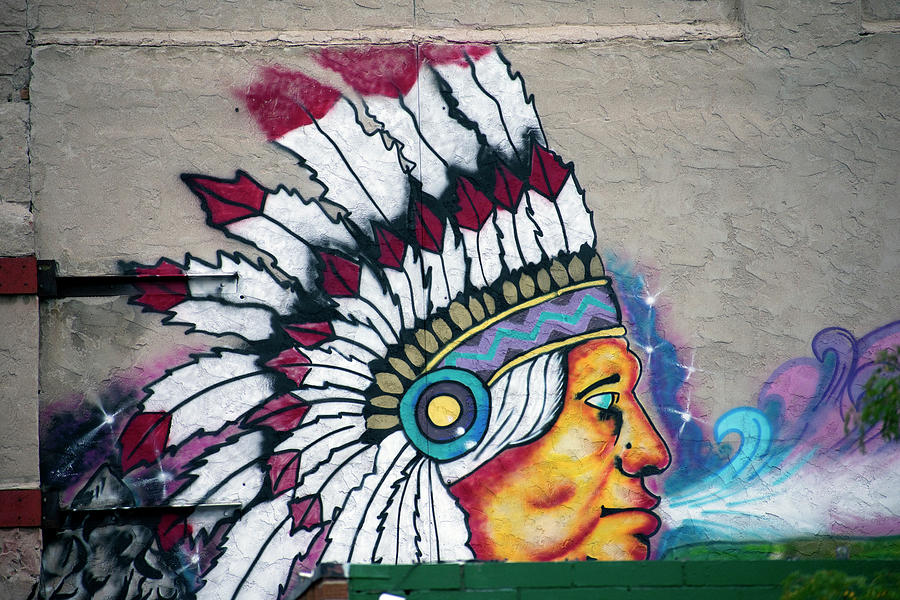The image showcases detailed outdoor wall art, prominently featuring a traditional Native American chief painted on a weathered, tan-colored building that appears aged and lined with grooves. The chief has brown skin, white hair, and visible wrinkles, indicating his elder status. He sports a traditional headdress adorned with red and white leaves arranged in multiple rows around a blue band. His expressive face, characterized by a large nose and a vivid blue eye, gazes off to the right side. Below the headdress, there's a zigzag pattern incorporating blue, purple, and yellow hues. Surrounding the chief are swirls of blue, violet, and white, which resemble stars or blowing wind emanating from his mouth. The artistic backdrop creates a dynamic scene, accented further by what appears to be a mountainous landscape behind him.